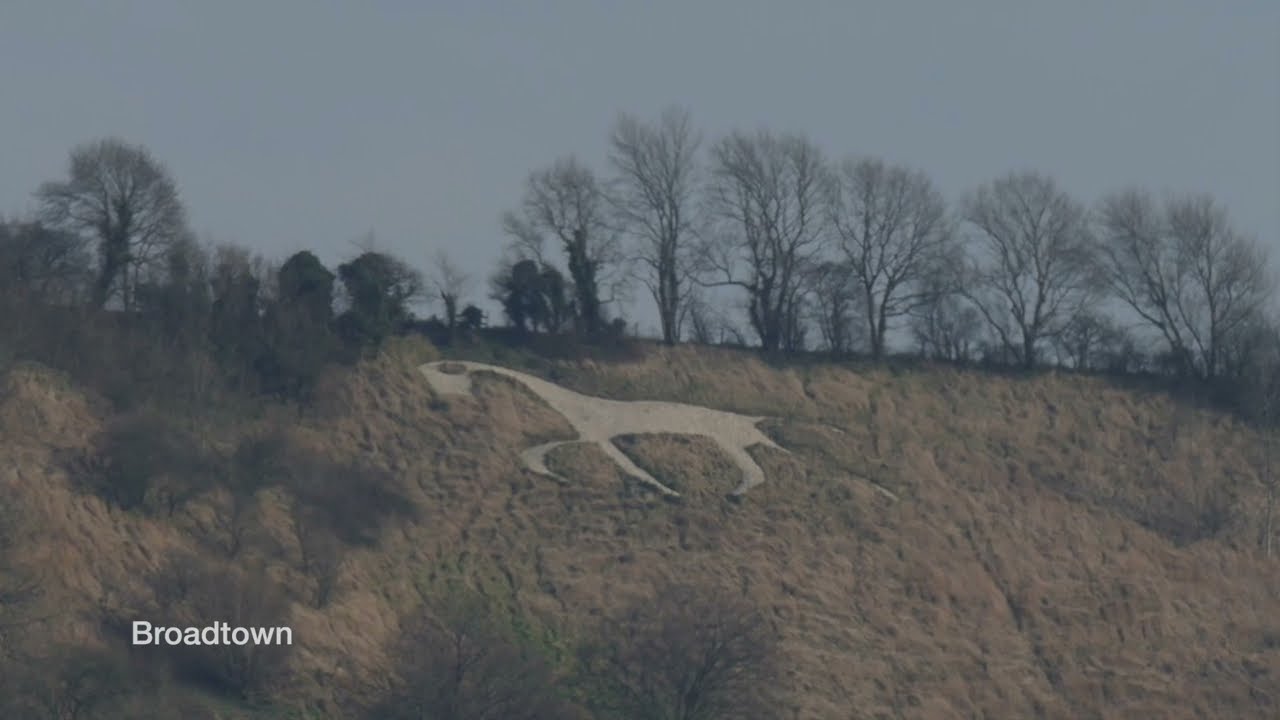The image captures an outdoor scene dominated by a large, steep hill covered in grass, bushes, and a mix of bare and leafy trees. The sky overhead is a dull grayish blue, contributing to the overall somber mood of the scene. A striking feature of the hill is a large, cutout silhouette of a horse, etched into the landscape, likely by removing grass down to the dirt, giving it an artistic appearance. Trees line the horizon at the top of the hill, adding depth to the setting. In the bottom left corner, the word "Broadtown" is displayed in white font. The image appears to have a slightly hazy or aged quality, suggesting it might have been taken in fall or early spring.